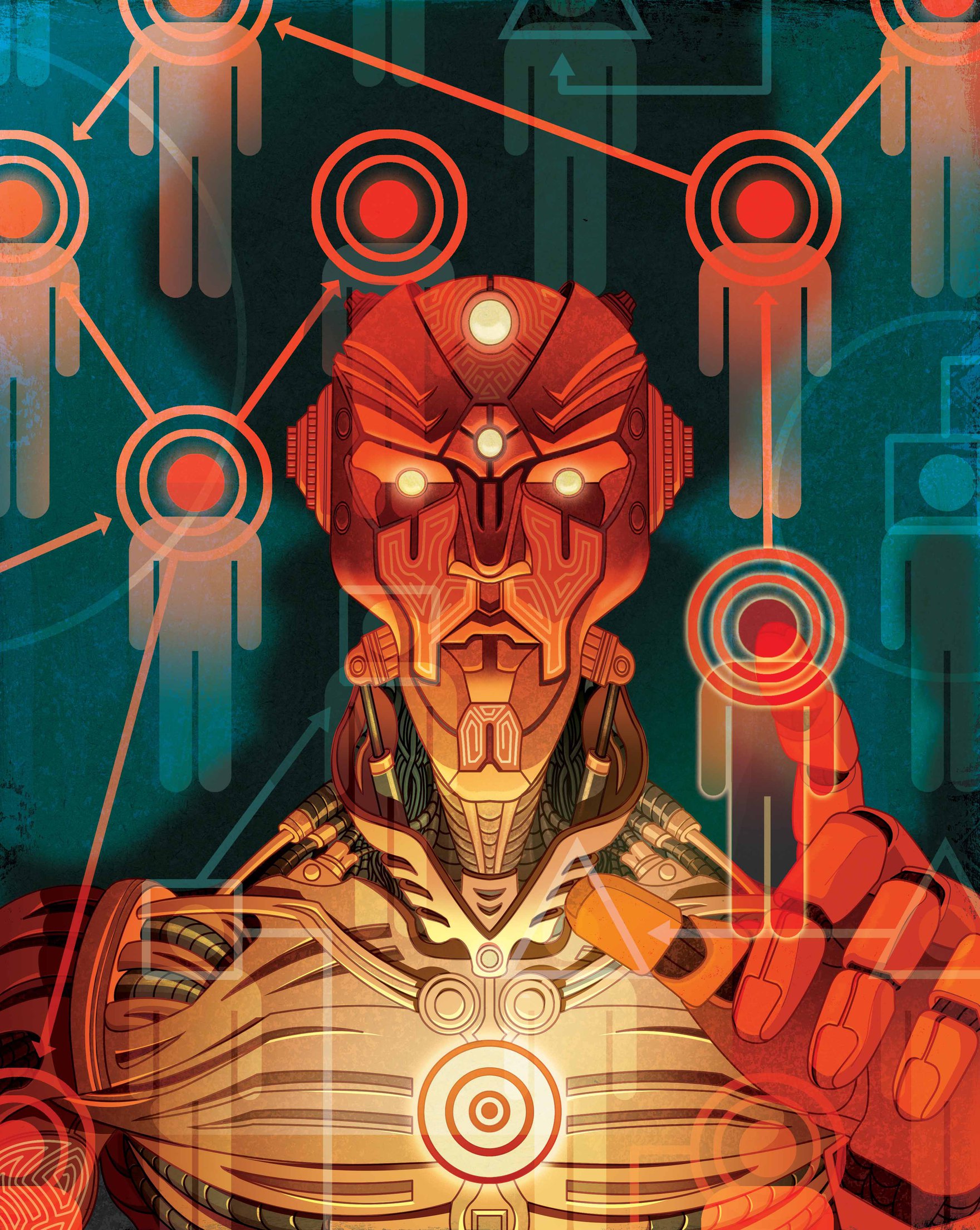The image is an abstract, almost cubist, computer-generated artwork featuring what appears to be a robotic or extraterrestrial being. The being is depicted in predominantly red-purple hues with a yellow-tinted lower portion. It possesses a human-like hand and fingers, adding a mechanical touch with oval-shaped appendages protruding from its chin and tiny cone-like ears. The head is colored reddish-orange with yellow dot eyes and a circular light on the forehead.

The chest area displays intricate lines resembling cables or scales, contributing to its robotic appearance, and features what seems like a shield, though it's challenging to delineate where the being's body ends and the armor begins. The background is dominated by a dark teal color with blue shades, adorned with patterns of men's restroom symbols, possibly floating or cloth-like, and red circles, adding to the scene's surreal nature.

The being's expression is serious, almost grimacing, and with its left hand, it engages with a translucent screen. The screen displays icons resembling the universal symbol for male, each with red circular heads and gray bodies. The being's touch activates a network of interconnected circles and lines, creating a web-like array of humanoid icons, emphasizing a strange, futuristic interaction.